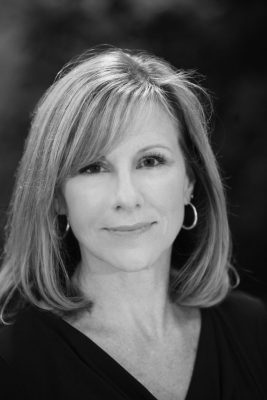This is a black and white head and shoulders photo of an attractive woman with brownish-blonde hair that falls to her shoulders. She has blondish hair with highlights and no bangs. Her eyes are dark but bright, and her eyelashes are long and well-groomed. She has thin eyebrows and small, barely visible ears. The woman is wearing medium-sized hoop earrings and a black top with a V-neckline, which isn't too deep. She has a perfectly proportionate nose and a slight, warm smile on her face, suggesting she is in her late 30s or early 40s. The background of the image is black, with some vague, unidentifiable whitish shapes around the edges. She is looking directly at the camera, exuding a familiar yet universally appealing presence.